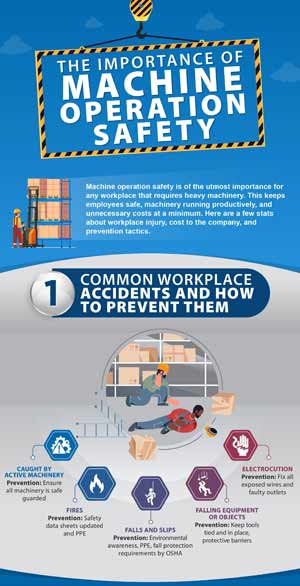The image is a workplace safety sign focused on machine operation safety. The poster features a blue background with a white lower half, bordered by an orange and black striped frame, giving the appearance of a wall hanging. The header reads, "The Importance of Machine Operation Safety." Below, a section titled “Common Workplace Accidents and How to Prevent Them” features various safety tips and prevention methods.

Illustrations include a cartoon man who looks like he fell, positioned near some boxes with a hard hat beside him, indicating fall-related accidents. There’s also an image of someone operating a forklift. Small text explains the significance of workplace safety, preventative measures, and associated statistics, but the print is too small to read clearly. Key highlighted safety topics include preventing accidents from active machinery, fires, falls, falling objects, and electrocution. Each type of accident is paired with specific prevention strategies, such as ensuring machinery is safeguarded, updating safety data sheets, using PPE (Personal Protective Equipment), and fixing exposed wires. 

The design's top and bottom borders are blue, while much of the critical text appears in gray, making the detailed safety guidelines challenging to read from a distance.